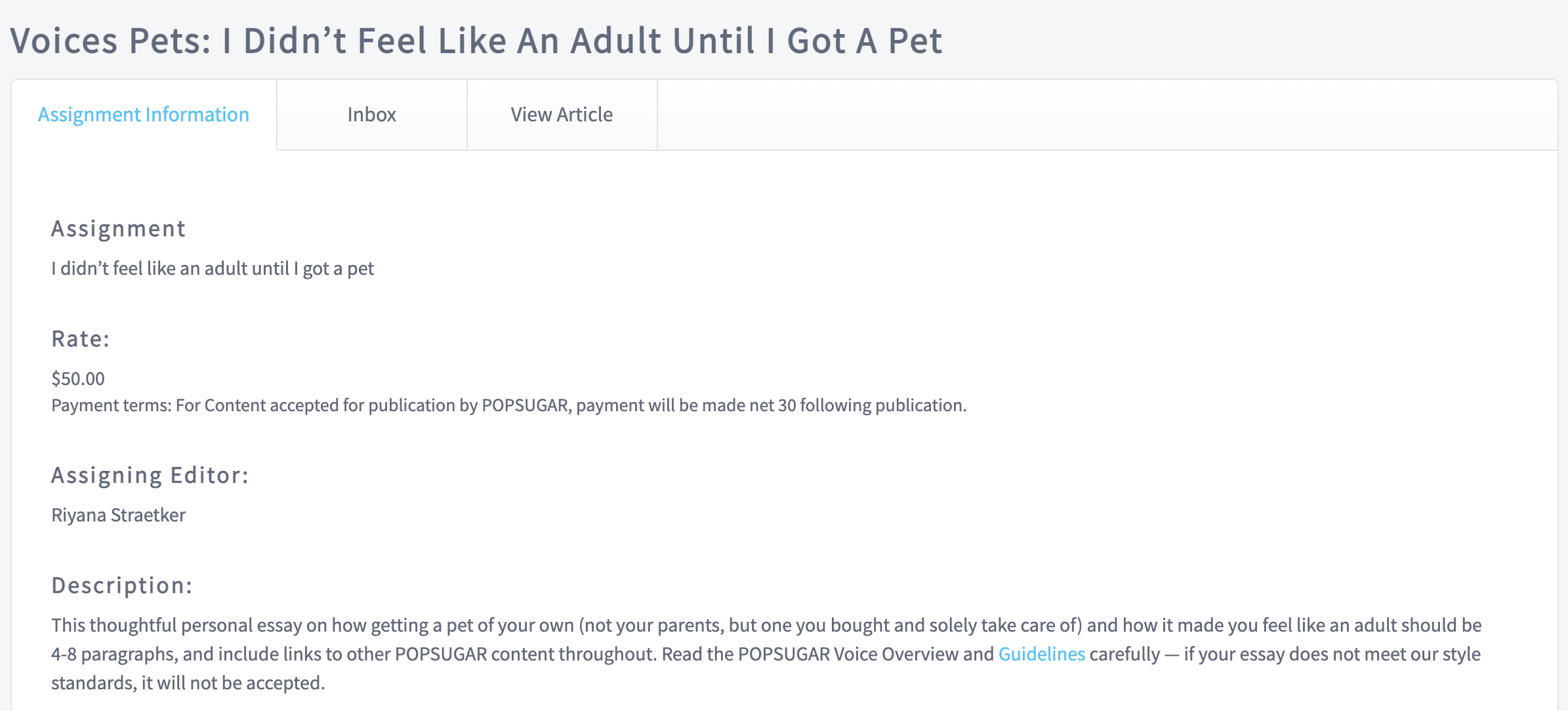**Detailed Caption:**

This image is a screenshot, potentially capturing a part of a website or someone's work inbox, specifically focusing on an assignment instruction page. The top section prominently features the heading "Voices; Pets: I Didn't Feel Like an Adult Until I Got a Pet," with each word capitalized. 

Beneath this header, the interface is divided into three tabs labeled "Assignment Information," "Inbox," and "View Article." The "Assignment Information" tab is highlighted in bright blue, indicating that it is the selected tab. 

In the main content area of the "Assignment Information" section, there is a white space containing text. The text displayed is as follows:

- **Assignment:** "I Didn’t Feel Like an Adult Until I Got a Pet."
- **Rates;** "$50."
- **Payment terms:** "For content accepted for publication by PopSugar, payment will be made net $30 following publication."
- **Assigning Editor;** "Rihanna Stryker."
- **Description;** "This thoughtful personal essay on how getting a pet of your own (not your parents, but one you bought and solely take care of) made you feel like an adult should be 4-8 paragraphs and include links to other PopSugar content throughout. Read the PopSugar voice overview and guidelines carefully—if your essay does not meet our style standards, it will not be accepted."

The entire text is set against a white background, providing a clear and uncluttered view of the assignment details.